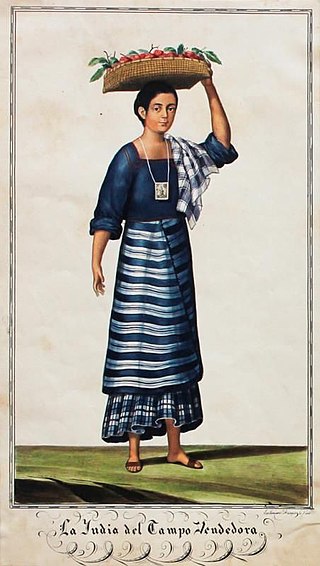In the image, we see a vibrant color painting of a Hispanic woman standing on a green surface. She is balancing a square basket filled with green and red apples on her head with her left hand. The woman is dressed in a dark blue top with long sleeves rolled up to her elbows. A blue and white checkered scarf is draped over her left shoulder. She wears two skirts: an outer one featuring blue and white horizontal stripes, and an inner one with a blue and white checkered pattern. Her brown sandals further hint at her being outdoors. She has short black hair and a white necklace around her neck that features a photo. Beneath the image, the words "La Giudia del Campo Zen de Dora" are written.